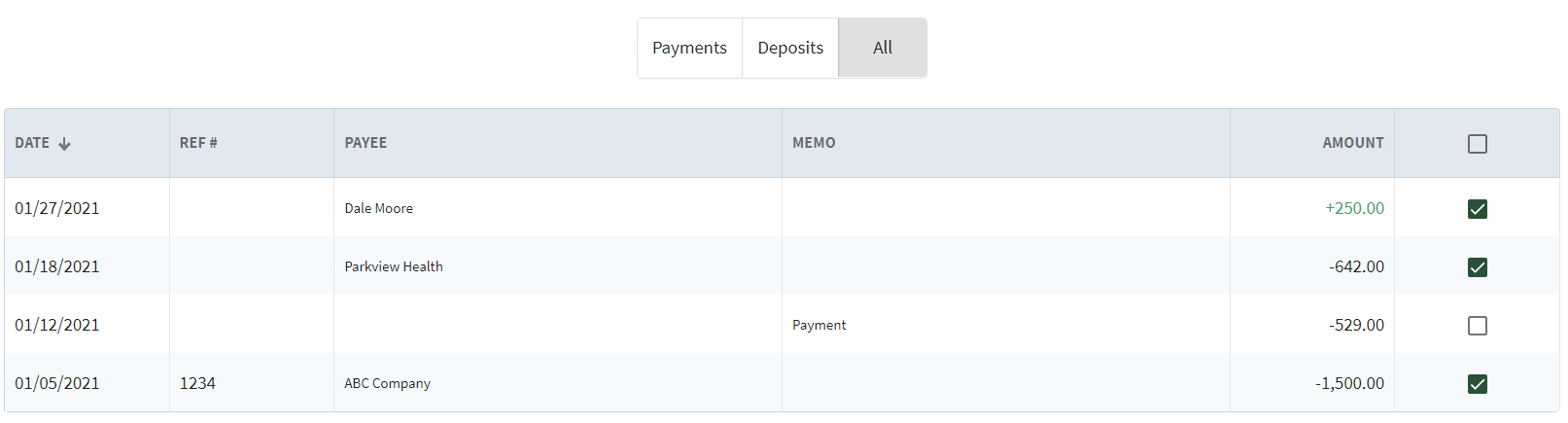This is an image displaying a financial management interface, likely a website or app, used for tracking and calculating expenses. At the top of the interface, there are three buttons labeled "Payments," "Deposits," and "All," with the "All" button highlighted in grey, indicating that the current table displays combined data from all categories.

Below these buttons, a table is presented with a header bar featuring a greyish background. Each column is clearly labeled: Date, Reference Number, Pay, Memo, Amount, and a tick box for selection. The rows in the table alternate between a white and a light grey background for better readability.

The entries in the table are as follows:
1. The first entry is dated January 27, 2021. There is no reference number provided. The payee is Dalemore with no memo information. The amount is a credit of $250 (+$250), and the checkbox is selected, indicating that this entry has been acknowledged or processed.
2. The second entry is dated January 18, 2021. Again, there is no reference number. The payee is Parkview Health with no memo information. The amount is a debit of $642 (-$642), and this entry is also checkmarked.
3. The third entry is dated January 12, 2021. There is no reference number or listed payee. The memo field notes "Payment," and the amount is a debit of $529 (-$529). This checkbox for this entry is not selected, suggesting it might not have been processed or acknowledged yet.
4. The fourth and final entry at the bottom of the table is dated January 5, 2021. The reference number for this one is 1234, the payee is ABC Company, and the memo field is empty. The amount is a significant debit of $1500 (-$1500), and its checkbox is selected.

This detailed table allows for careful tracking and review of financial transactions, making it easy to monitor and manage expenses and income.